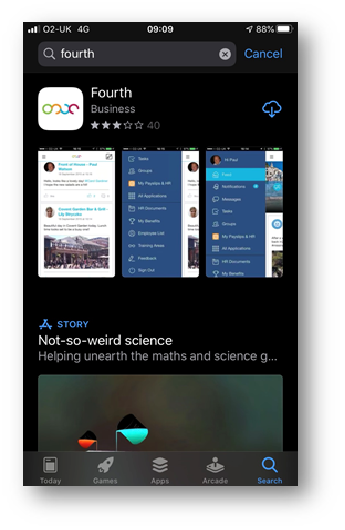This is an image capturing a mobile screenshot from the Google App Store, specifically showcasing the business app named "Forth." The app currently holds a rating of 3 out of 5 stars across 40 reviews. The screenshot was taken at 3:09, with the device battery level at 83%, indicated at the top of the screen.

In the detailed view of the app, there are three distinct screenshots displayed. The first screenshot shows the main interface of the app with a clean white background. The second screenshot provides more details about the app, particularly highlighting the functionality and design of the left pane. The third screenshot zooms in on this left pane, which has a blue background. There is accompanying text that reads, "It's not so weird science helping unearth the maths and science."

The app's avatar features a simple yet colorful design with a white background. It consists of four semicircles aligned in a row, each differing in color from left to right: green, orange, blue, and an inverted red U-shaped semicircle.